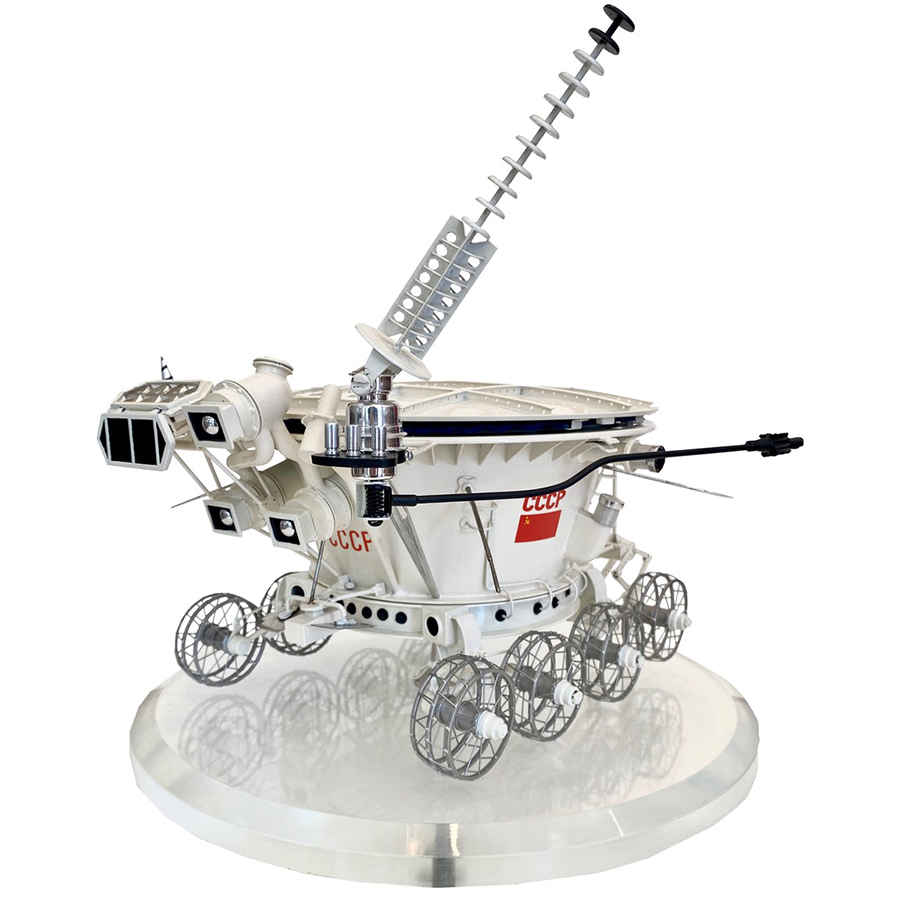The photograph captures a detailed image of a contemporary robotic instrument set against a stark white background, allowing its features to be clearly observed. The robot, round and predominantly white, is positioned on a round, clear base that may also function as a mirror, enhancing the visibility of its details. It is equipped with four meshed metal wheels on each side, resembling air fans. Prominently, the letters "CCCP" are emblazoned in red on both the side and the back of the machine. Additional elements include a large metal rod with an attached black rod, various small boxes with imprints, and a distinctive antenna featuring round circular disks. A small red rectangle is also visible on the body beneath the "CCCP" lettering, adding to the machine's intricate design.